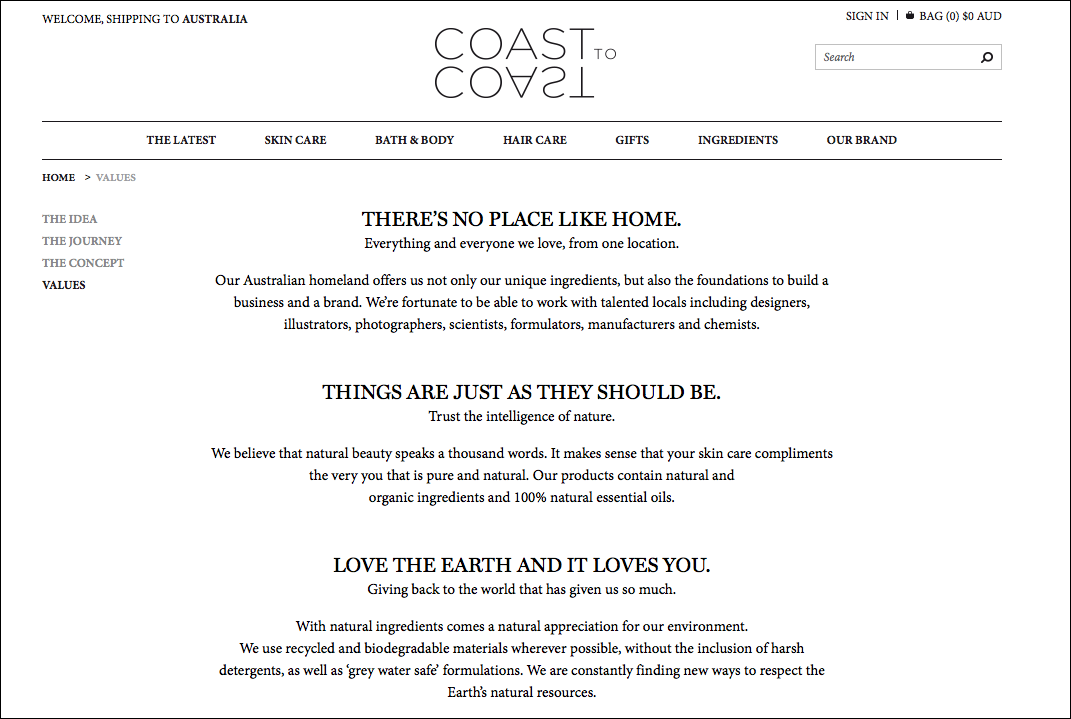Here is a cleaned-up and detailed caption for the described image:

---

Screenshot of the Coast2Coast website homepage. At the top left corner, it features the text "Welcome, shipping to Australia" alongside an "OK" button. On the top right, there are options to "Sign In," an icon of a shopping bag labeled "Bag (0)" indicating an empty shopping cart, and total spending displayed as "$0 AUD."

Below these options lies a search bar with an accompanying magnifying glass icon for searching the website. Centrally positioned and prominent, the Coast2Coast logo is displayed in full capitals. The "COAST" text appears with a mirrored reflection below it and a distinctive "2" placed alongside in the format "T-O."

Beneath the logo, there are two horizontal rules guiding the navigation to various sections of the site: "The Latest," "Skin Care," "Bath and Body," "Hair Care," "Gifts," "Ingredients," and "Our Brand." 

On the left sidebar, a breadcrumb navigation shows "Home > Values." The sidebar also lists subsections in gray text: "The Idea," "The Journey," "The Concept," and prominently highlighted, "Values."

The main content area elucidates three core values of the brand: "There is no place like home," "Things are just as they should be," and "Love the Earth, and it loves you." Below these values, expandable text provides further details, reinforcing the brand's commitment to these principles.

---

This caption comprehensively describes the layout and key elements of the Coast2Coast website homepage, capturing the navigation structure, branding, and thematic messaging.